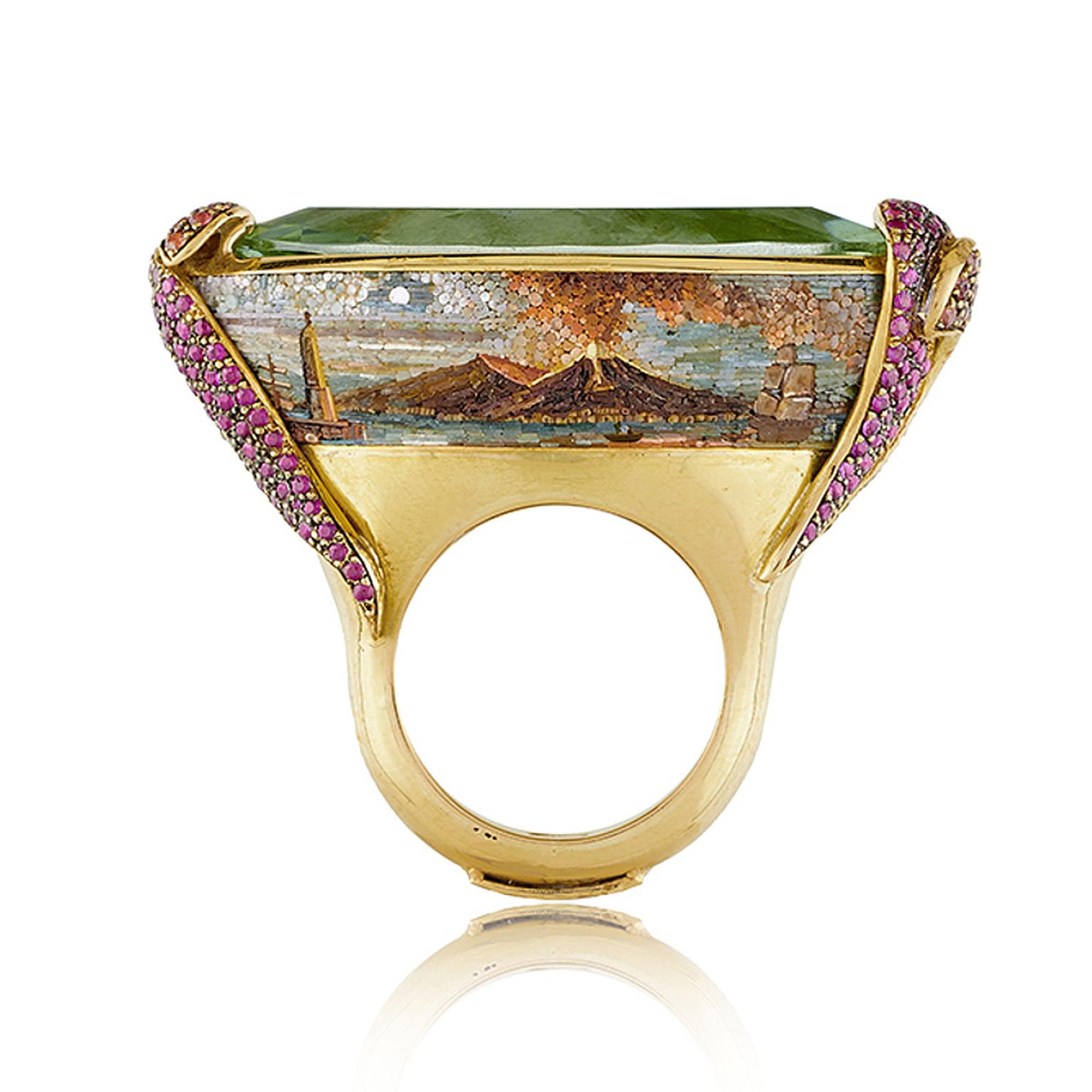This up-close photograph showcases an ornate and intricate gold ring, meticulously designed with extraordinary detail, likely for a product listing. The gold band encircles the finger, and the ring stands prominently high. At its base is a miniature, intricately painted scene of an erupting volcano, flanked by what appear to be demolished buildings. The sides of the ring feature gold snake heads, resembling cobras, each set with purple gemstones. These serpents rise up and support a large, flat-topped green gem, possibly jade or emerald, which crowns the ring. The gem is oblong with slanted sides, making the ring extend about an inch off the finger. This unique piece is both artistic and striking, likely serving as an extraordinary piece of jewelry for display or sale.